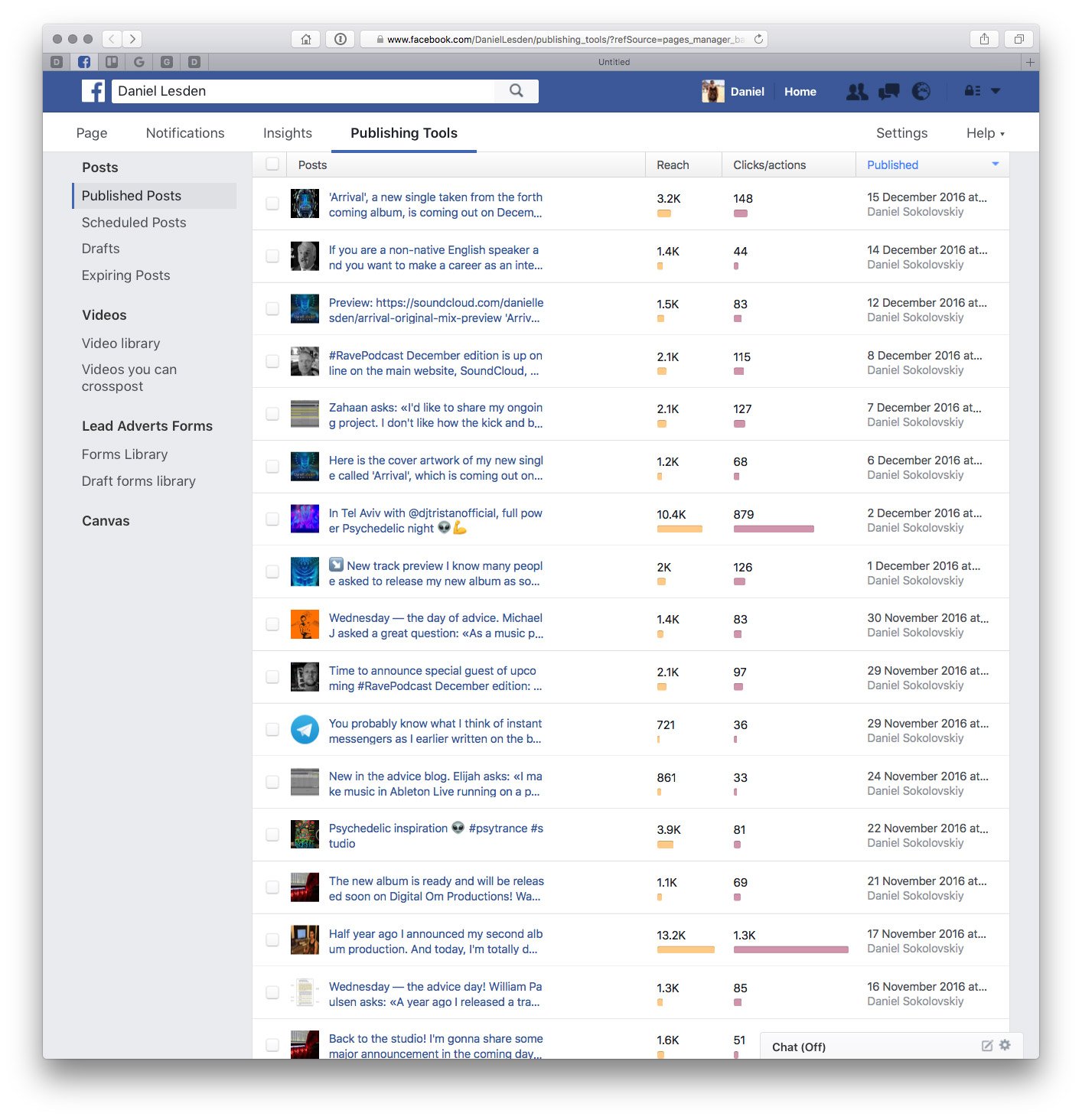This detailed image captures an old Facebook page interface, showcasing a variety of elements and a series of posts by Daniel Sokolovsky. At the top, there’s a green task bar containing the search field, populated with the URL “www.facebook.com/DanielNeston/publishing_tools/?NE1source=pages_manager”, next to a reload button. The header also includes navigation icons for Home, People, Chat, Notifications, and a settings menu with a down arrow.

Directly below, there are tabs for Pages, Notifications, Insights, and Publishing Tools. On the left side, a sidebar lists options like Posts, Published Posts (highlighted), Scheduled Posts, Drafts, Expiring Posts, Videos, Video Library, Videos You Can Post, Lead Ad Forms, Forms Library, Draft Forms Library, and Canvas.

The main content area features a collection of posts by Daniel Sokolovsky, each detailed with metrics on reach, clicks, and actions. The posts include:

1. **Arrival:** A new single from an upcoming album, set to release in December. 
   - Metrics: 3.2k reach, 148 clicks/actions
   - Date: December 15, 2016

2. **Career Advice for Non-Native English Speakers:**
   - Metrics: 1.4k reach, 44 clicks/actions
   - Date: December 2016

3. **Preview of "Arrival":** Link to SoundCloud preview.
   - Metrics: 1.5k reach, 83 clicks/actions
   - Date: December 2016

4. **Rave Podcast:** Predictions available on SoundCloud.
   - Metrics: 2.1k reach, 115 clicks/actions
   - Date: December 2016

5. **Original Ongoing Project:** 
   - Metrics: 2.1k reach, 127 clicks/actions
   - Date: December 2016

6. **Cover Artwork for "Arrival":**
   - Metrics: 1.2k reach, 68 clicks/actions
   - Date: December 2016

7. **Tel Aviv Event with DJ Tristan:** 
   - Metrics: 10.4k reach, 87 clicks/actions
   - Date: December 2016

8. **New Track Preview:**
   - Metrics: 2k reach, 126 clicks/actions
   - Date: December 2016

9. **Advice from Michael J:** 
   - Metrics: 1.4k reach, 83 clicks/actions
   - Date: November 2016

10. **Special Guests Announcement for Rave Podcast:** 
    - Metrics: 2.1k reach, 97 clicks/actions
    - Date: November 2016

11. **Opinion on Instant Messages:** 
    - Metrics: 721 reach, 36 clicks/actions
    - Date: November 2016

12. **Advice by Black Elijah:** 
    - Metrics: 861 reach, 33 clicks/actions
    - Date: November 2016

13. **Psychedelic Inspiration Post:** 
    - Metrics: 3.9k reach, 81 clicks/actions
    - Date: November 2016

14. **Announcement of New Album:** 
    - Metrics: 1.1k reach, 69 clicks/actions
    - Date: November 2016

15. **Announcement of Second Album:** 
    - Metrics: 13.2k reach, 1.3k clicks/actions
    - Date: November 2016

16. **Year-Past Release Anniversary:** 
    - Metrics: 1.3k reach, 85 clicks/actions
    - Date: November 2016

17. **Studio Update:** Upcoming major announcement.
    - Metrics: 1.6k reach, 51 clicks/actions

To the right of the main post area, a chat tab appears labeled "chat off," indicating an inactive chat feature. 

This comprehensive view highlights Daniel Sokolovsky's active engagement and detailed analytics for each post on his historical Facebook page.